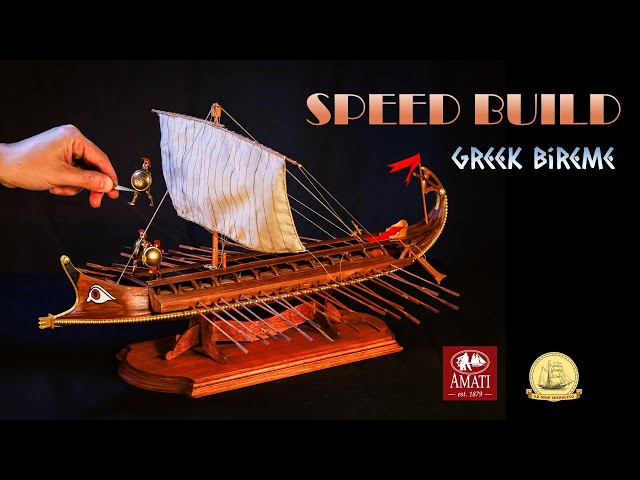The image depicts the front of a box for a model ship, likely a Greek bireme but resembling a Viking warship with its detailed craftsmanship. The background of the box is entirely black, accentuating the ship's features: a single square white sail with numerous strings supporting the mast, and long oars extending from the hull. The ship itself is made of wood, with a carved eye on the left side of the bow, indicating its historical design. The deck of the ship is medium brown, and the display base is a rich cherry wood color.

Several miniature soldiers or toy pirates with shields are positioned on the deck, suggesting an ancient, battle-ready scene. Additionally, a human hand, using tweezers, is in the midst of placing another small figurine onto the ship, highlighting the intricate, hands-on nature of the model building process.

Text elements are prominently displayed across the box. On the right side, it reads "Speed Build" in orange, uppercase letters, along with "Greek Bireme" (sometimes misspelled as "Barim"). On the lower part of the box, there is a gold logo featuring a sailboat, and to the left of this, a red box with white text that states "Amadi, established 1879." These elements reinforce the product's branding and historical authenticity.